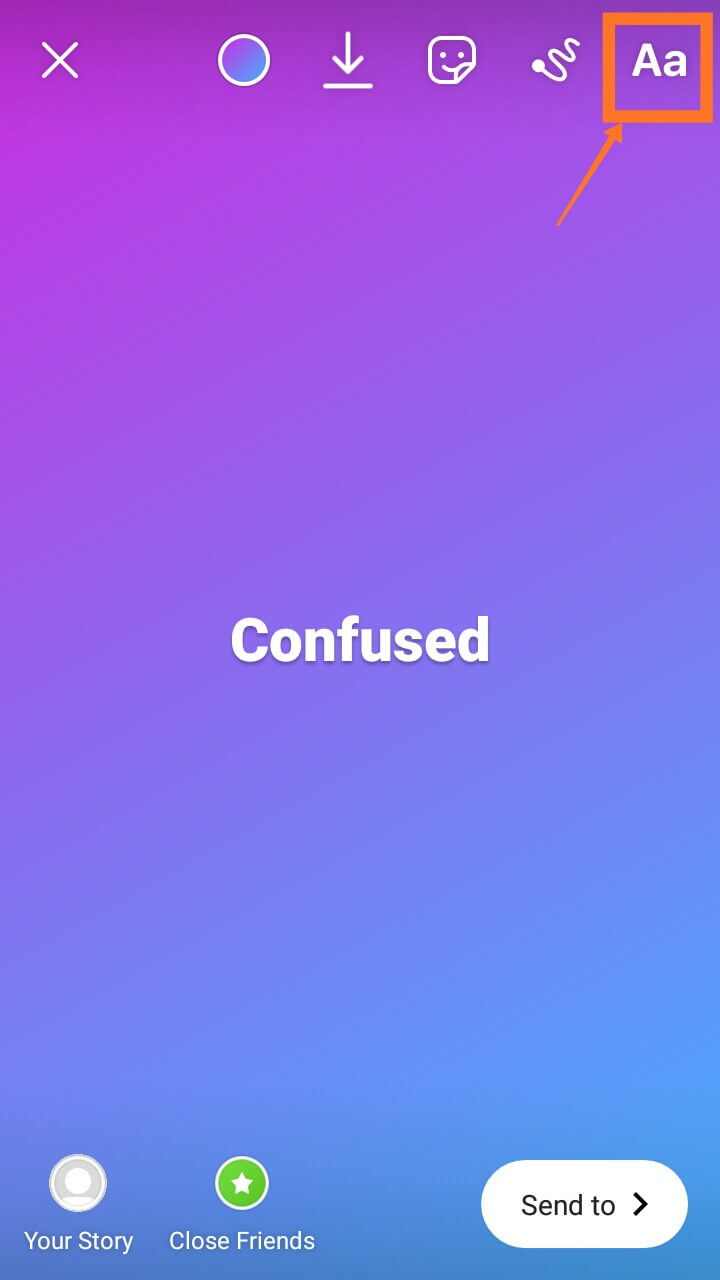In this image, we observe what appears to be a user interface of an app. Dominating the top right corner, there's a vibrant orange square enclosing a capital 'A' and a lowercase 'a', both rendered in white. Adjacent to this square, an orange arrow extends from the bottom left, further emphasizing it. Moving leftward along the top right, there's a small white squiggly line, a sticker featuring a smiley face, a downward-pointing arrow, and finally, a circle filled with a gradient of blue and purple hues.

On the top left corner sits a white 'X', likely serving as a close button. Centrally positioned within the image, the word "confused" stands out in bold white text, capturing attention. Transitioning to the bottom right, there's a white rectangular button labeled "send to," accompanied by a rightward-pointing arrow.

In the bottom left corner, there are two options: "your story" and "close friends." Above each label rests a corresponding circle. The circle above "close friends" is particularly notable, featuring a green background with a white star emblem centered within it.